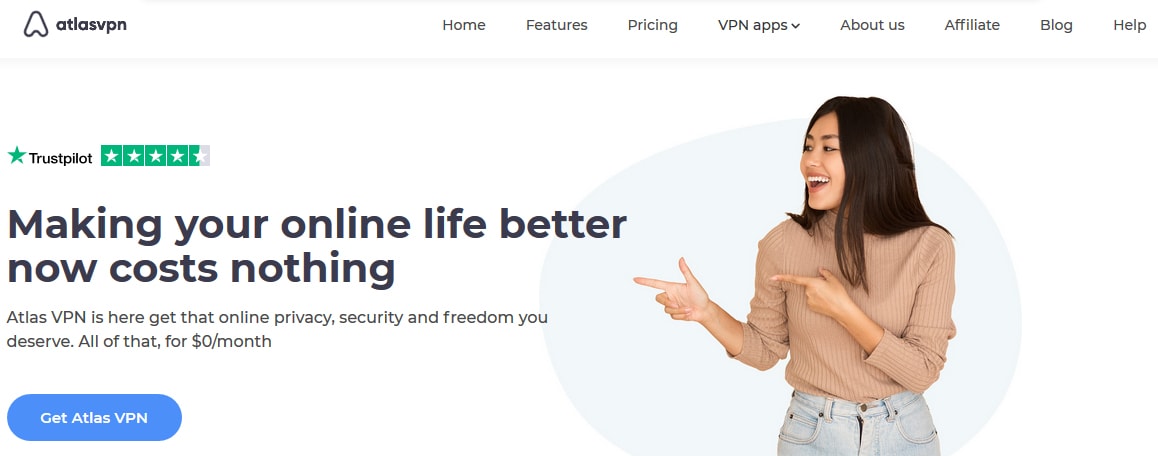The homepage of the Atlas VPN website features a clean, minimalistic design with a primarily white color scheme that is both empty and aesthetically appealing. At the top left, the Atlas VPN logo is displayed prominently, followed by the name "Atlas VPN." The top menu comprises various options including Home, Features, Pricing, VPN Apps (with a dropdown menu), About Us, Affiliates, Blog, and Help.

Central to the page, there is a stock image of a smiling Asian woman pointing towards the website's main motto. The motto reads: "Making your online life better now costs nothing." Directly above this motto, Trustpilot's badge showcases a 4.5-star review, adding credibility to the service.

Below the main motto, another slogan asserts, "Atlas VPN is here. Get the online privacy, security, and freedom you deserve. All of that for $0 a month." Concluding the message is a prominent call-to-action button that says, "Get Atlas VPN."